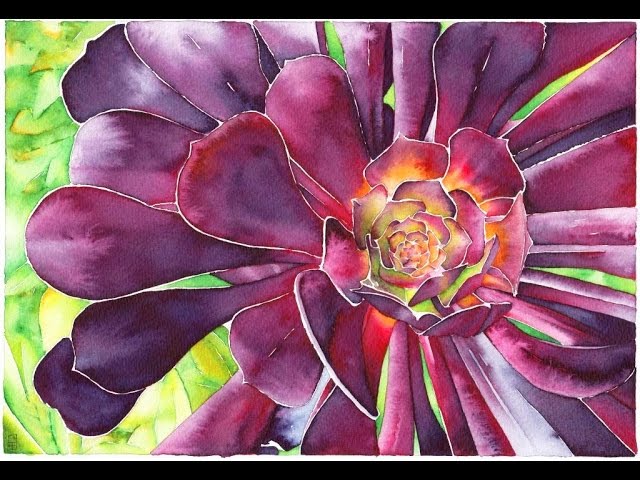This is an extremely detailed watercolor painting on a wide canvas, bordered at the top and bottom by thin black bars with a white line just above and below the main painting. The centerpiece of the artwork is a large flower with many petals, arranged in a big circular shape. The outermost petals are a darker, rounded purple with skinnier tips, and the very tips of these petals are white. As the petals move inward, they transition to a lighter grape-like purple.

The innermost petals create a spiraling pattern with changing colors starting from a lime green at the center and blending into orange and purple. This gives the middle of the flower a rose-shaped or lotus-like appearance. Surrounding the flower are abstract green leaves, adding to the depth and realism of the piece, although it's clear that this is a work of graphic art rather than a photograph. The painting's attention to detail and vibrant color transitions make it both mesmerizing and realistic in its portrayal of nature.